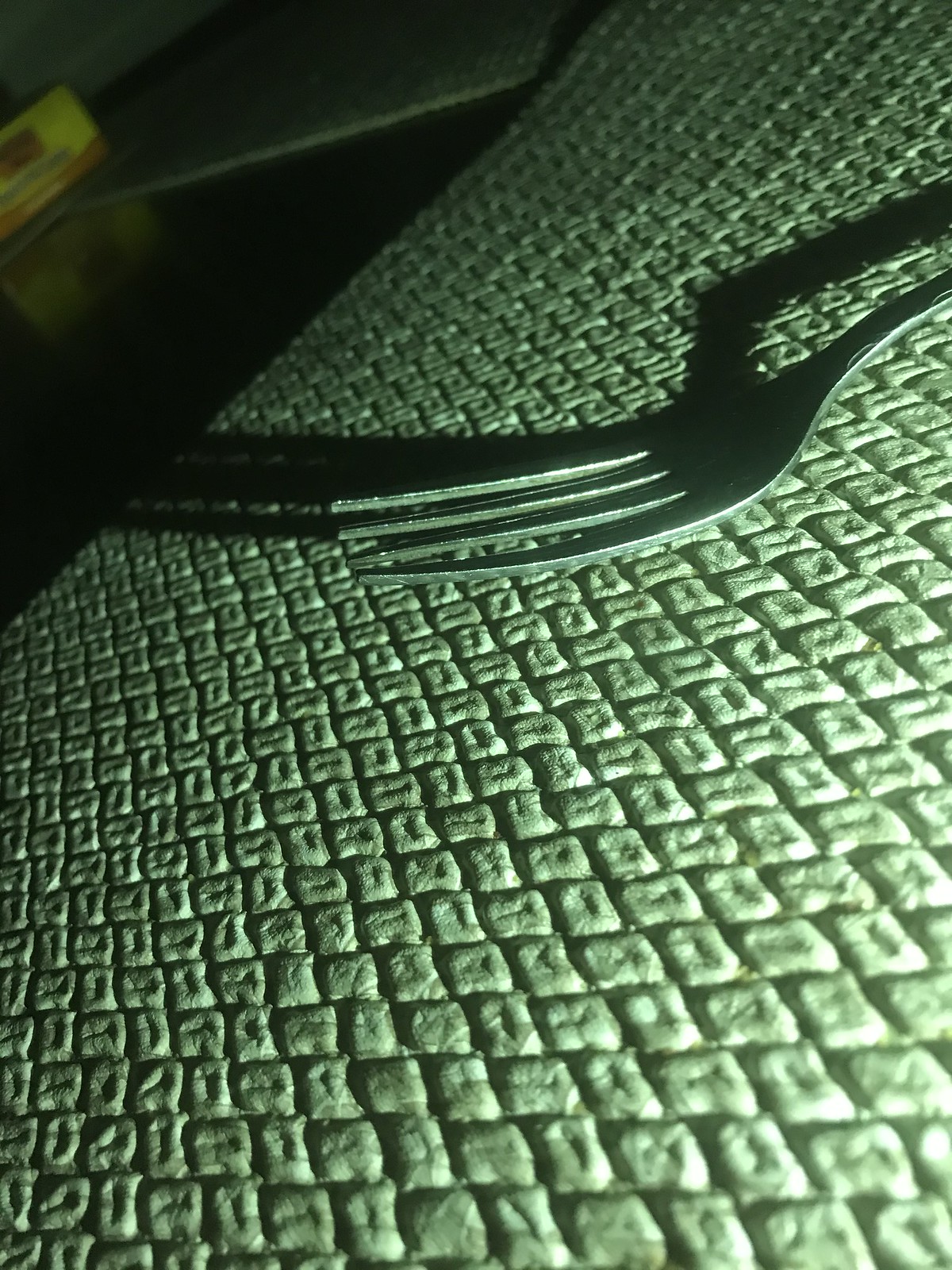In this dramatic, close-up photograph, a green plastic fork rests on a green checked mat with a textured design, featuring small square bumps. The limited light source, emanating dimly from the bottom right corner, casts stark, elongated shadows of the fork's tines and handle across the mat, emphasizing the texture and creating a sense of depth. The fork itself is partially visible, with only the tines and a sliver of the handle shown, lying towards the upper center right of the image and facing left. The dark surroundings obscure many details, although vague, blurry shapes in the background hint at another mat and an out-of-focus container, possibly white with red markings. The overarching darkness of the scene, coupled with the focused illumination, lends the image a dramatic and almost mysterious atmosphere.